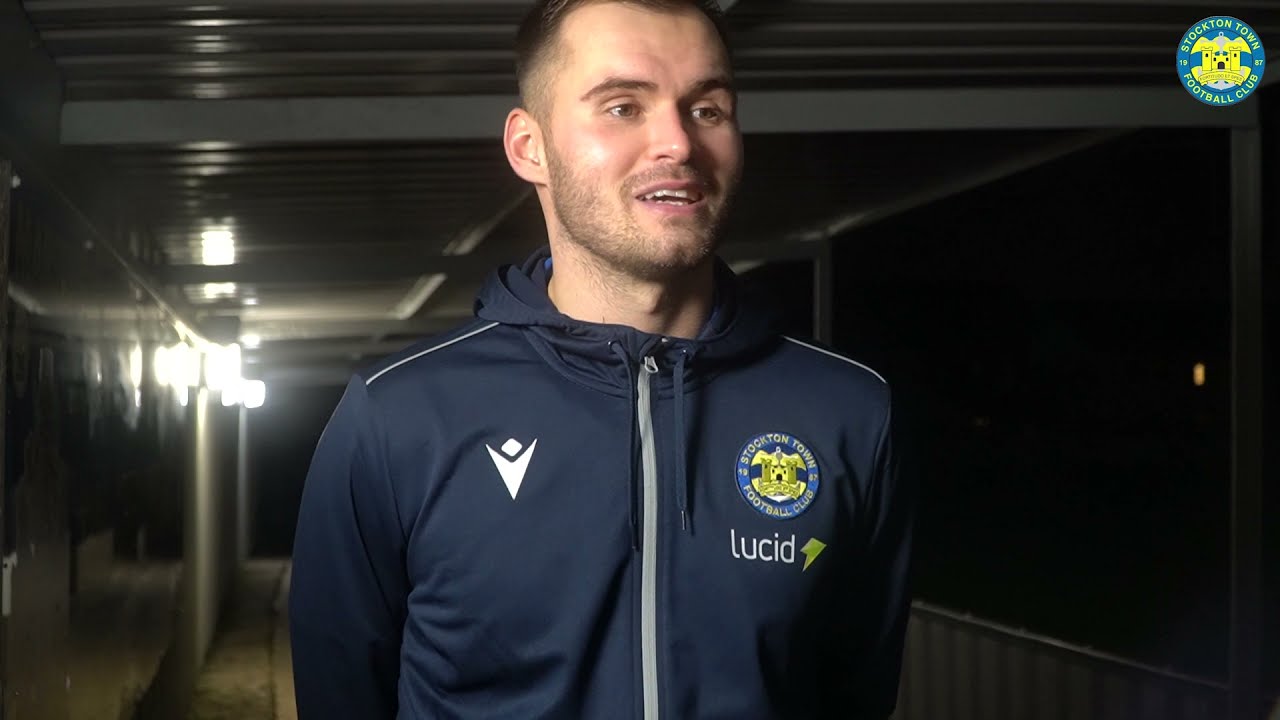In this detailed photograph, a white man, likely an athlete in his late 20s to early 30s, stands prominently in the middle of an outdoor corridor-like space under a flat metallic roof. The background, pitch black and seemingly empty with distant lights, suggests a nighttime scene. The man, presenting a scrubby stubble beard, is adorned in a dark blue hoodie or zip-down jacket, which appears slightly shiny. Prominently displayed on the chest area of his jacket are several logos, one of which reads "Lucid." Beneath this logo, the text "Stockton Town Football Club" indicates his affiliation as a football player. The man gazes slightly to his right, his mouth slightly open as though mid-sentence, perhaps engaged in conversation or an interview. Adding to the atmosphere, a blue and yellow logo of the Stockton Town Football Club is visible in the top right corner of the frame.